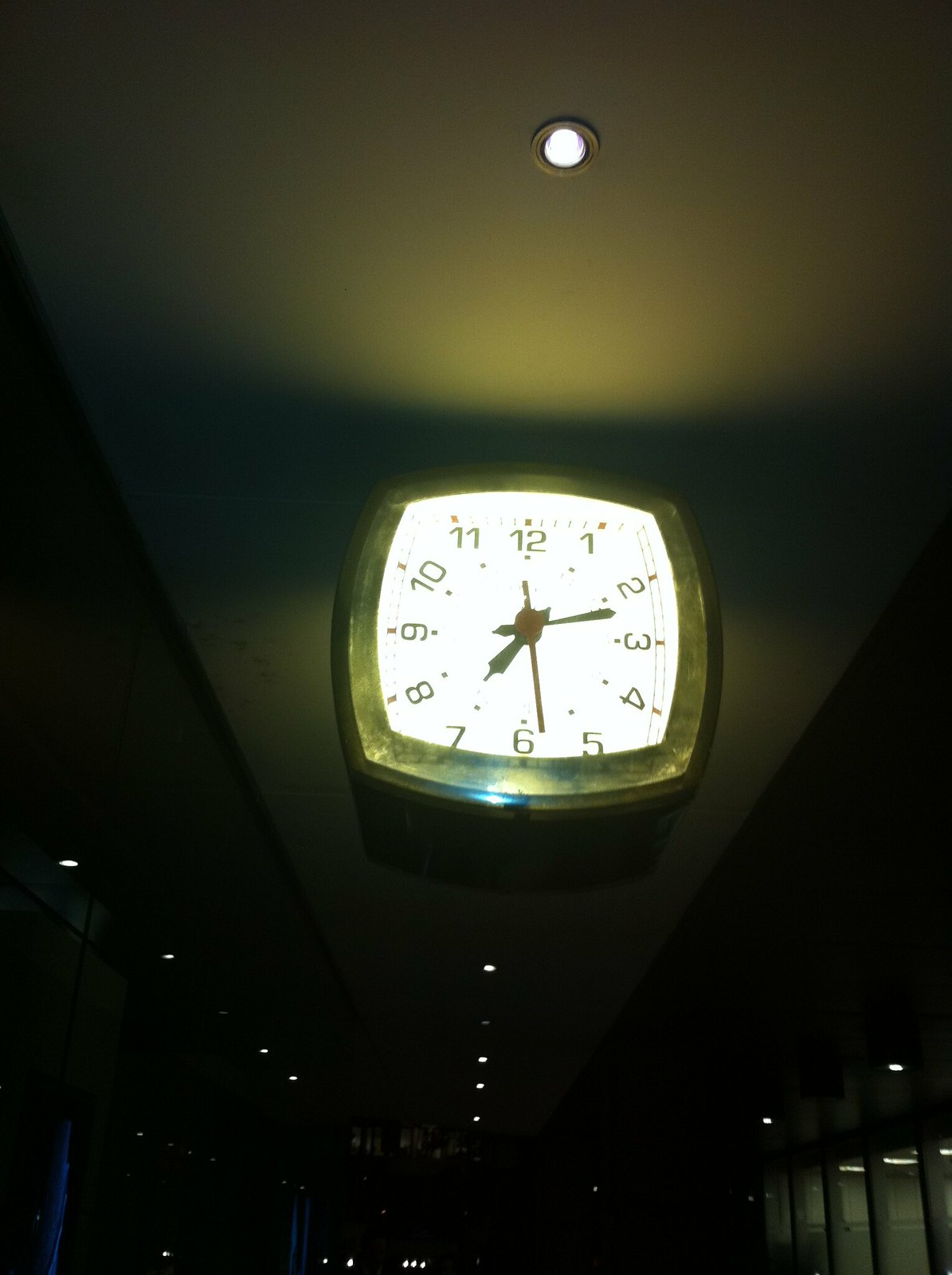This image features a large, elegant clock with backlighting mounted on the ceiling of a dimly lit hallway. The clock is not perfectly square; its shape resembles a square attempting to morph into a circle, with gently curved edges. The face of the clock displays Arabic numerals, and its hands indicate the time is around 7:12 p.m., with the small hand on the 7, the long hand between 2 and 3, and the second hand near 6. The clock has a golden or faux-gold finish, contributing to its striking presence. The setting appears to be a dark building, likely at night, evoking a moody atmosphere with minimal lighting except for the clock's illumination and a few scattered, circular ceiling lights extending throughout the hallway. A conference room is faintly visible to the right, and another ceiling light closer to the viewer is also in focus, enhancing the image's somber and quiet ambiance.